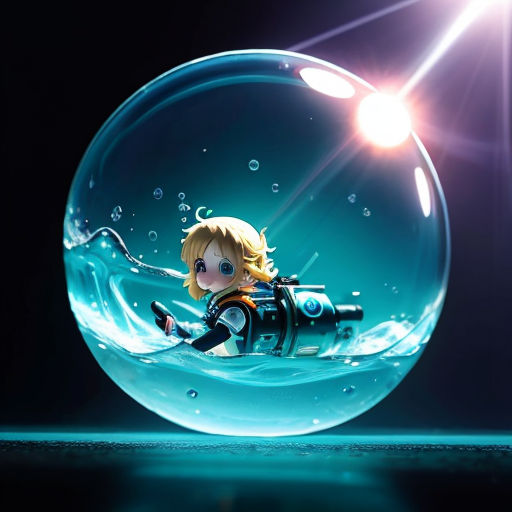This digital artwork features a clear, see-through globe or sphere with a sunbeam shining down and reflecting off it from the upper right, all set against a pitch-black background. Encased within this crystal-like globe is an anime or video game-style young girl with blonde hair and large eyes. She is dressed in light battle gear and has an intricate, large contraption on her back, resembling a space suit sans helmet. The lower half of the globe is filled with water, enveloping the girl up to her waist, and creating splashes and bubbles around her. Though the globe appears to be positioned on a surface, only a hint of the table is visible.